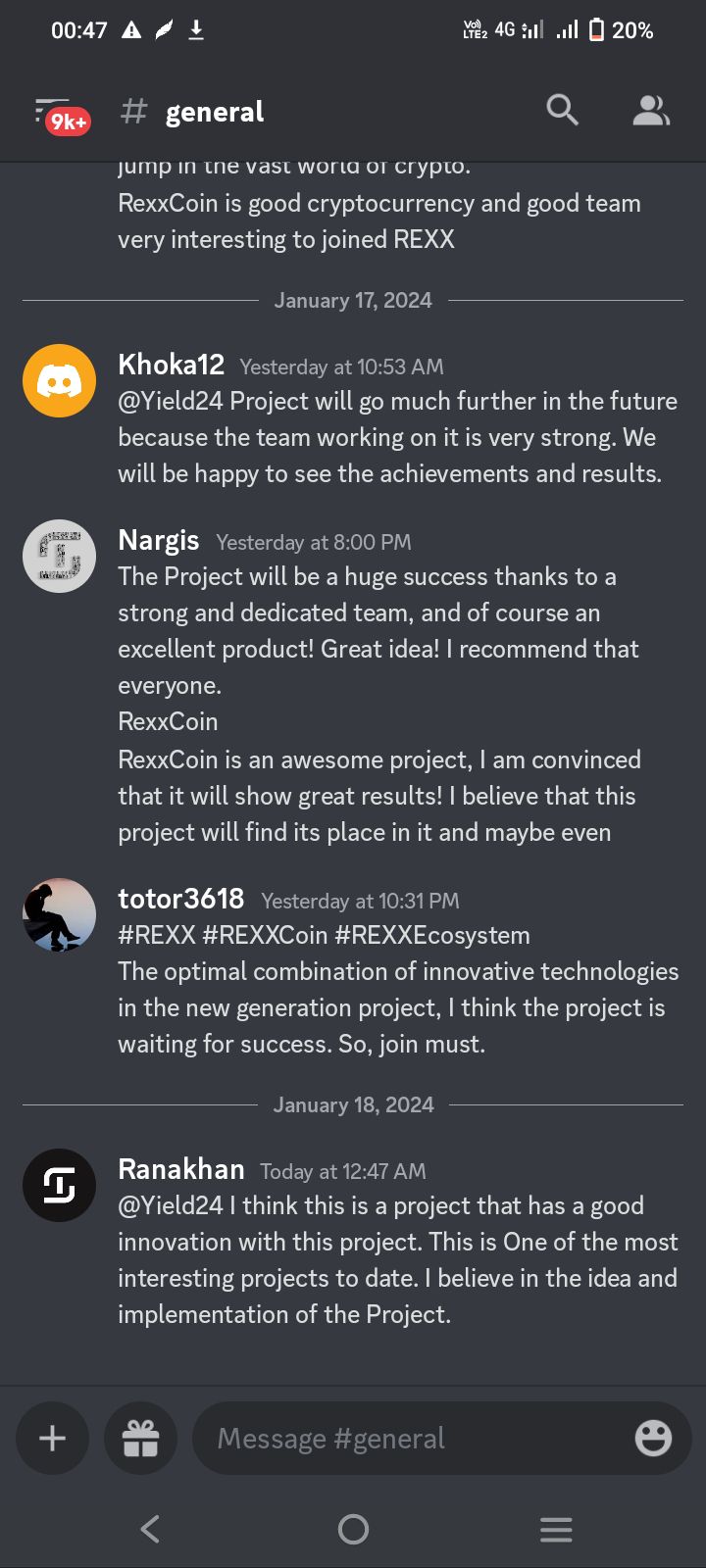A detailed caption for the image could be:

"A screenshot captured from a smartphone shows a project discussion within an app. The phone's status bar at the top indicates it is 00:47 AM, on a 4G network with three bars, not connected to Wi-Fi, and with a 20% battery level. The app's interface features a gray background with white text and has a header bar displaying '#general' in gray. On the left, there is an icon of three horizontal lines accompanied by '9K' encircled in red. On the right, there is a search magnifying glass icon and a profile button depicted as a silhouette of a person. At the bottom of the screen, the phone's navigation menu is visible, including a left-pointing arrow, a circle, and another three-line horizontal menu button. Within the app, various threads from different users are discussed. Each user is represented by an icon, the first being yellow with a video game controller. The conversation includes replies, mentions (denoted by '@'), and numerous hashtags, focusing on a topic called 'Rexcoin.'"